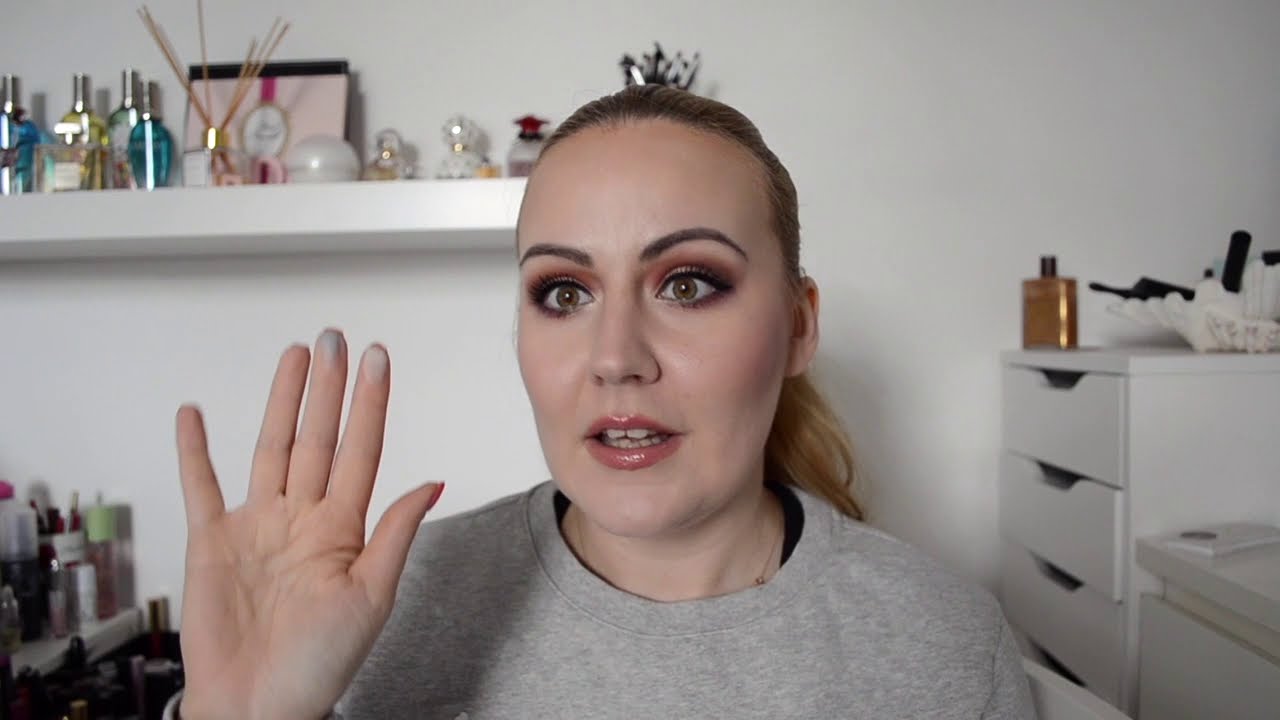The image is a close-up photograph of a Caucasian woman, around 25 to 30 years old, with a somewhat shocked expression on her face as she gazes slightly to the left of the viewer. She has wide brown eyes accentuated with purple eyeshadow, and she's wearing pink lipstick. Her blonde hair is neatly pulled back into a low ponytail. Clad in a gray sweatshirt with a black t-shirt peeking underneath, she raises her right hand, palm facing forward, as though making an oath.

The woman stands against a white backdrop, which includes a floating white shelf on her left. This shelf holds numerous perfume bottles, a reed diffuser, and other personal care items. To her right (the left side of the viewer), a white dresser with closed drawers is visible, topped with a distinctive golden bottle with a black cap and other indistinct items. The scene suggests a bedroom or personal space, meticulously organized and serene in its white decor.